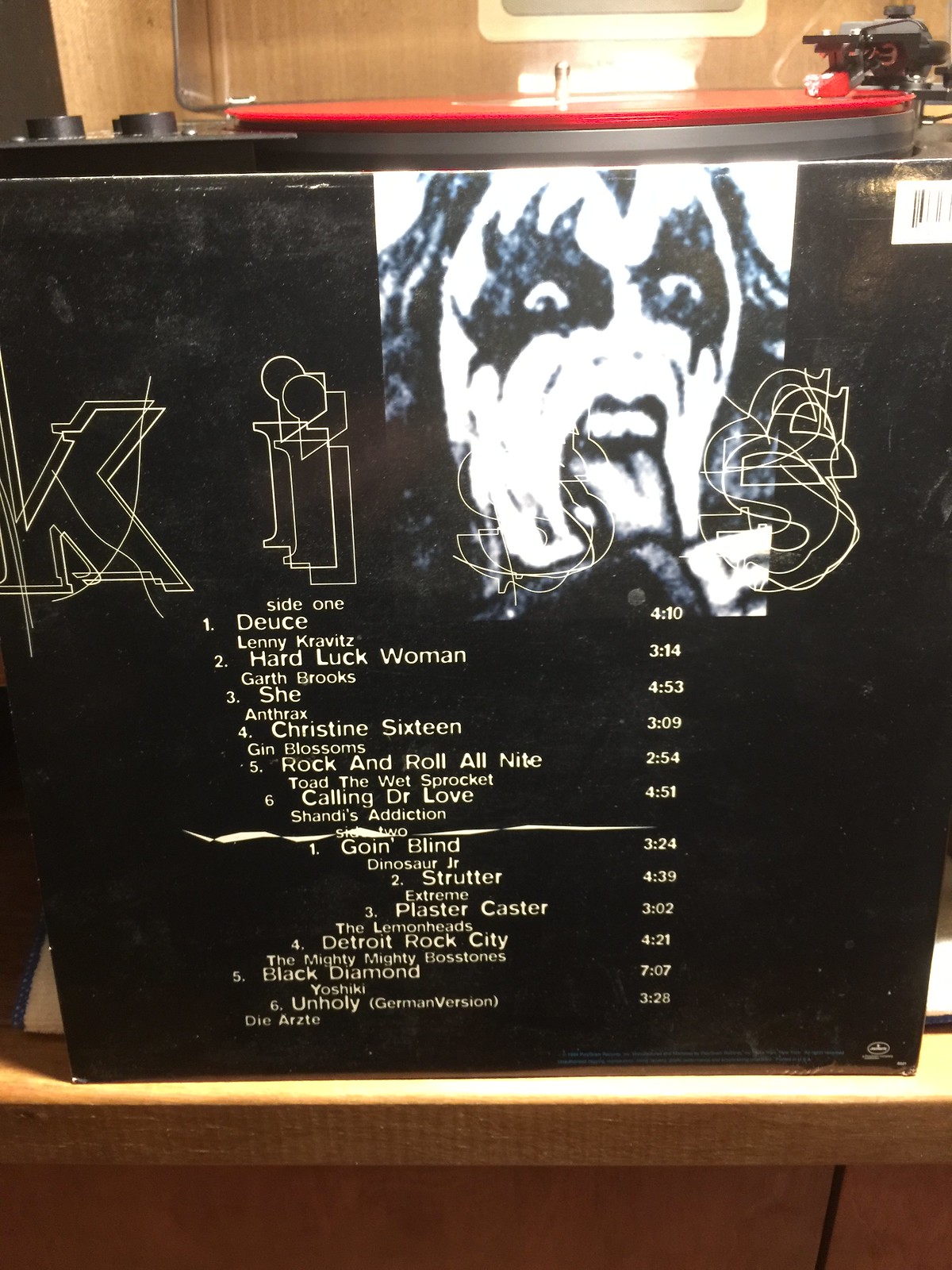The photograph is of a vintage turntable resting on a wooden plinth, playing a red-colored vinyl record. Positioned in front is an album cover with a black background, featuring the iconic makeup-clad face of a KISS band member in the top right corner. The face is heavily adorned with black makeup around the eyes, resembling a mask, while the rest of the face is predominantly painted white with black accents. The figure has dark, flowing hair that is cropped out of the frame, and a long, gray nose with a gradient of white and black paint.

The album cover prominently displays the word "KISS" overlaying the image of the band member. Surrounding this are faint listings of various songs, which are covers of KISS tracks performed by other artists. Among these cover songs are "She" by Anthrax, "Detroit Rock City" by The Mighty Mighty Bosstones, and "Strutter" by Xtreme. Other song titles include "Deuce," "Hard Luck Woman" by Garth Brooks, "Christine 16," "Rock and Roll All Nite," "Calling Dr. Love," and "Shandy's Addiction."

The red vinyl record spinning on the turntable, alongside the visually striking album cover, evokes a sense of nostalgic admiration for classic rock and the legendary band, KISS. The turntable itself has two adjustment knobs visible behind it and is set against a wooden table or counter, with a backdrop that may be either a wood wall or the top of the record player, adding a rustic charm to the scene.